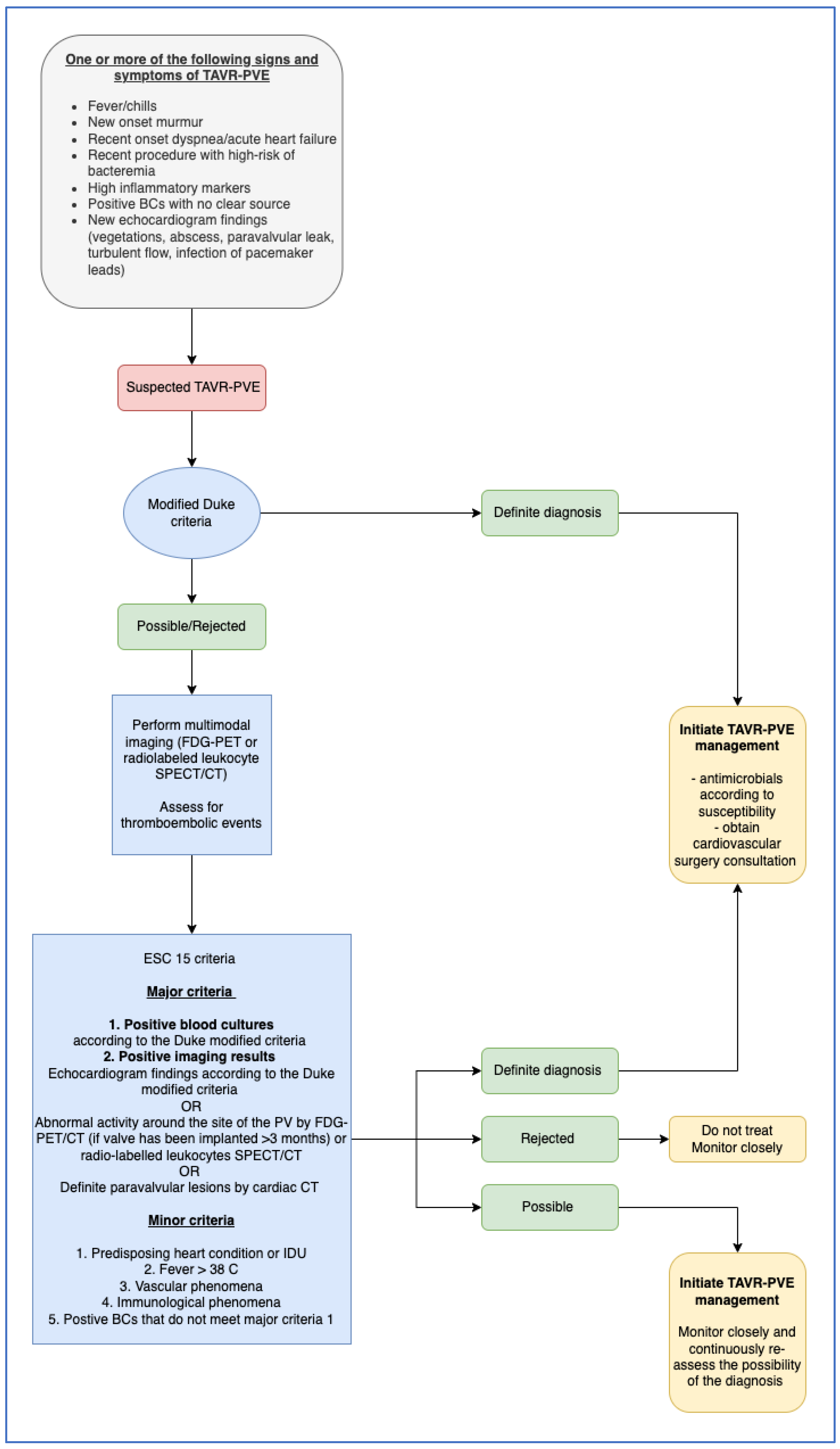The image features a detailed flowchart for diagnosing and managing TAVR-PVE (Transcatheter Aortic Valve Replacement-Associated Prosthetic Valve Endocarditis). Starting from the top, a white box states "one or more of the following signs and symptoms of TAVR-PVE," including fever, chills, new onset murmur, recent onset dyspnea, acute heart failure, recent procedure with high risk of bacteremia, high inflammatory markers, positive blood cultures with no clear source, and new echocardiogram findings such as vegetations, abscess, paravalvular leak, turbulent flow, and infection of pacemaker leads. An arrow leads down to a red box labeled "suspected TAVR-PVE," which then directs to a blue oval that says "modified Duke criteria."

From the modified Duke criteria, the flowchart branches into two paths: one leading to a definite diagnosis on the right, and another leading downwards to a possible rejection. After a definite diagnosis, the chart instructs to "initiate TAVR-PVE management." For a possible rejection, it says to "perform multimodal imaging, FDG-PET or radio-labeled leukocyte SPECTCT, and assess for thromboembolic events." 

The diagram also includes a section for the ESC-15 criteria under major and minor categories, which help further in the assessment. Depending on the results, the path leads back to either a continued diagnosis (which directs to initiate management) or a rejection, advising to "monitor closely." The flowchart is color-coded with sections in red, blue, green, and yellow, all featuring black text for clarity.